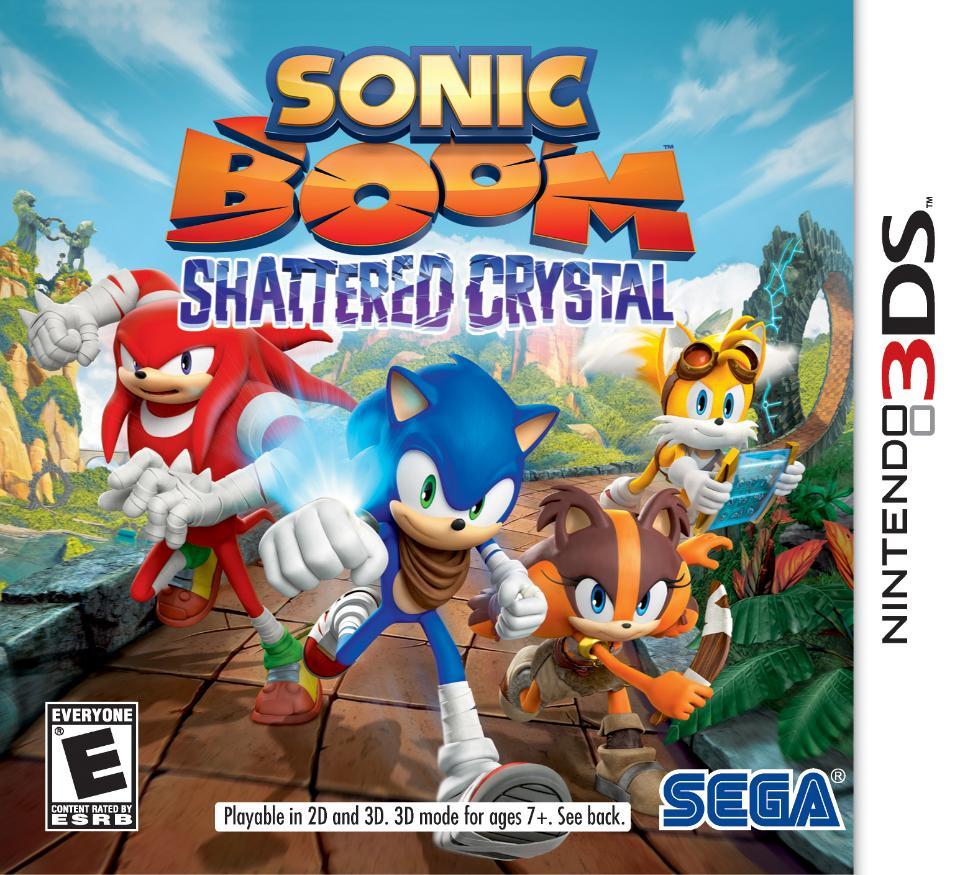The image is the cover of the video game "Sonic Boom: Shattered Crystal," designed for the Nintendo 3DS system, as indicated by the label on the right side. The game is produced by SEGA, whose logo can be found at the bottom right of the cover. Prominently featured are several characters running on a stone path set against a vibrant, tropical backdrop with trees, bushes, cliffs, and a mostly sunny sky with a few clouds. Sonic the Hedgehog, the iconic blue character with white gloves, leads the pack. To his left is a similar red creature also wearing white gloves. To Sonic's immediate right is a brown and orange creature resembling a fox or raccoon, wielding a wooden knife and sporting bear-like ears. Further to the right is Tails, the yellow fox flying with two tails and holding a chart. The game's title is prominently displayed, along with the rating "E for Everyone" by the ESRB, visible in a white rectangle on the bottom left. Additionally, there is black text at the bottom center specifying that the game is playable in 2D and 3D, with 3D mode suitable for ages seven and up, advising to see the back for more details.